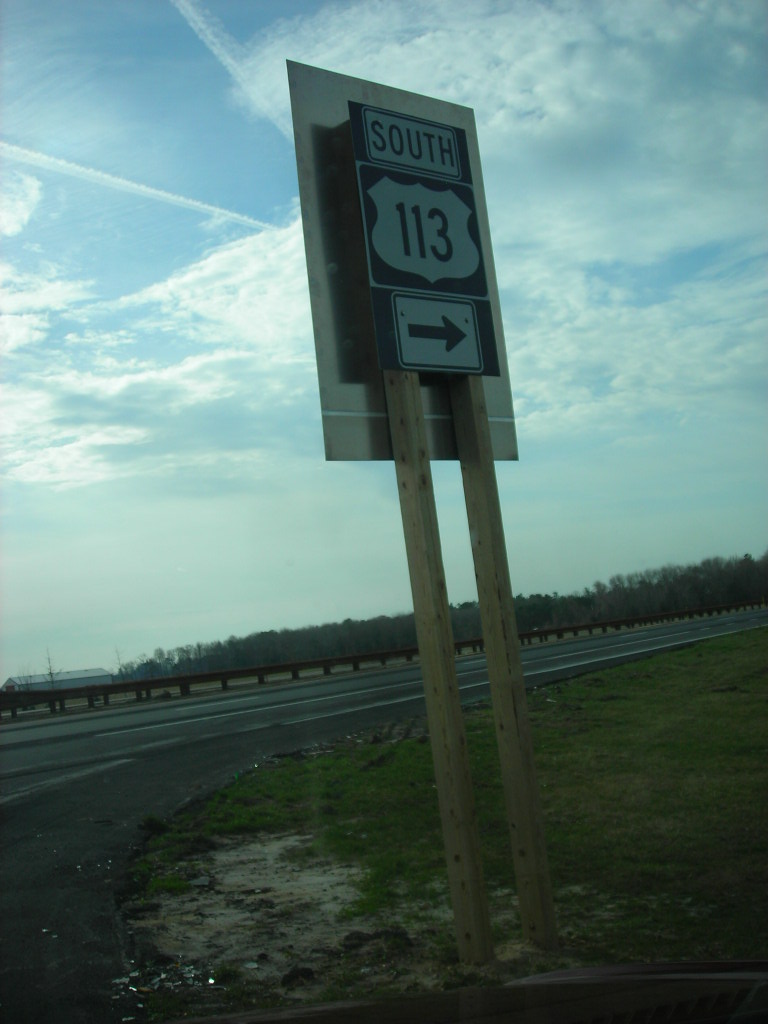The image depicts a highway street sign viewed from the perspective of someone sitting in a car, just having pulled up at an intersection. The sign, which is primarily green, has the word "South" at the top, with the number "113" prominently displayed below it. An arrow on the sign points to the right, indicating the direction of the highway. The sign is mounted on two sturdy wooden posts. 

In the foreground, patches of grass are visible to the right, leading up to the road that curves in that direction. The left side and the straight-ahead view are obscured, emphasizing the road turning right. The background consists predominantly of a clear blue sky accentuated with wispy white clouds. Beyond the immediate roadside, a cluster of trees occupies a small portion of the image, with what appears to be a barn or similar structure partially visible to the left of the trees. The composition captures a sense of open rural space, with the sky and the sign being the dominant features in the scene.